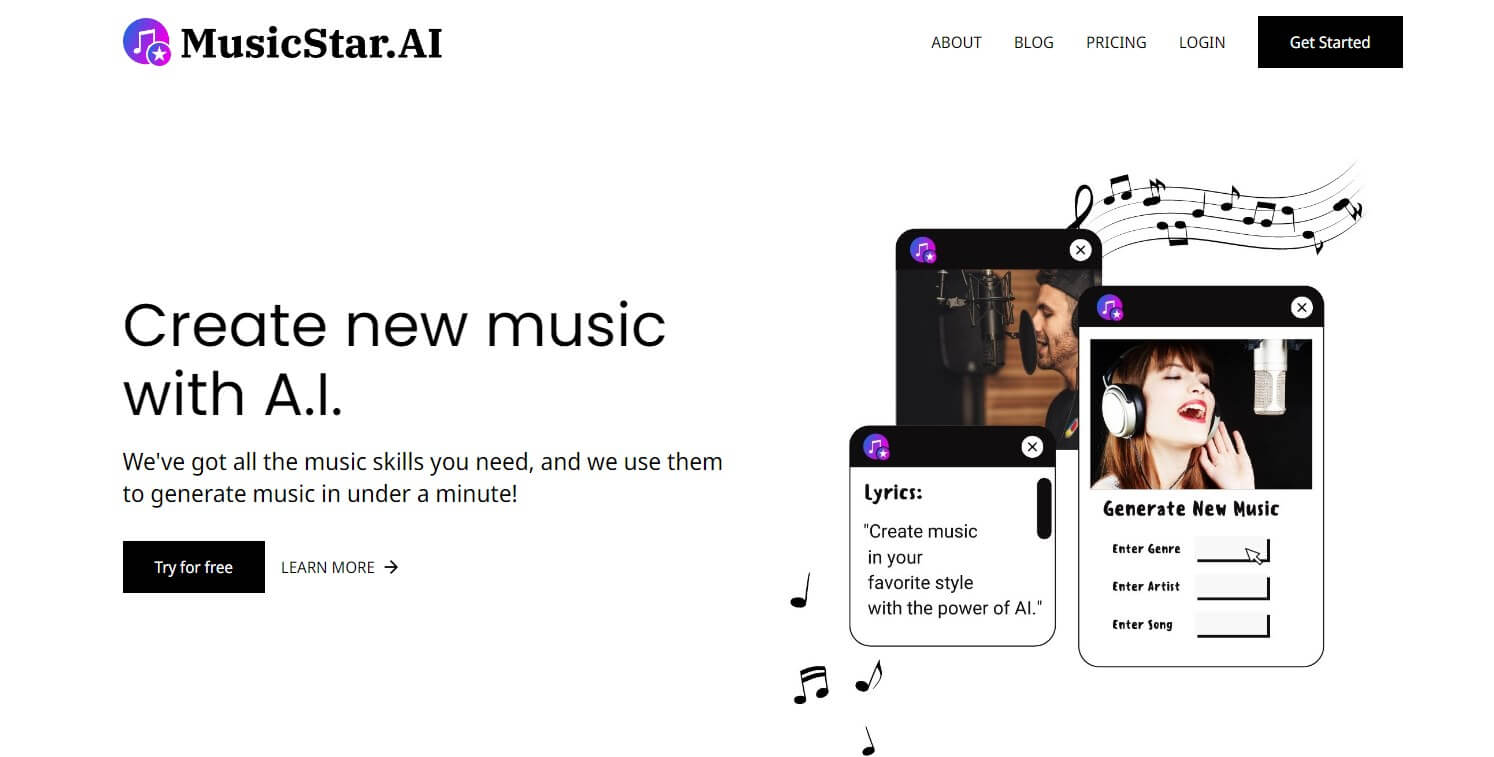**Caption:**

In this digital image representing MusicStar.ai, two individuals are engrossed in the act of singing, showcasing the platform's capabilities in music creation. 

On the left is a man, approximately 32 years old, with tan skin. He is passionately singing into a large microphone, almost the size of his face, capturing his dedication. 

To the right is a woman, around 25 years old, with fair skin. She wears headphones and sings into a microphone positioned just a few inches from her mouth, illustrating her immersion in the musical process.

The image is accompanied by a promotional text on the left side that reads: "Create new music with AI. We've got all the music skills you need and we use them to generate music in under a minute." 

Below the text are interactive elements including a "Try for Free" button, a "Learn More" link, and a "Get Started" button, along with navigation options such as Login, Pricing, and Blog.

MusicStar.ai encapsulates the harmony between human talent and artificial intelligence, offering users an innovative way to create music swiftly and effortlessly.